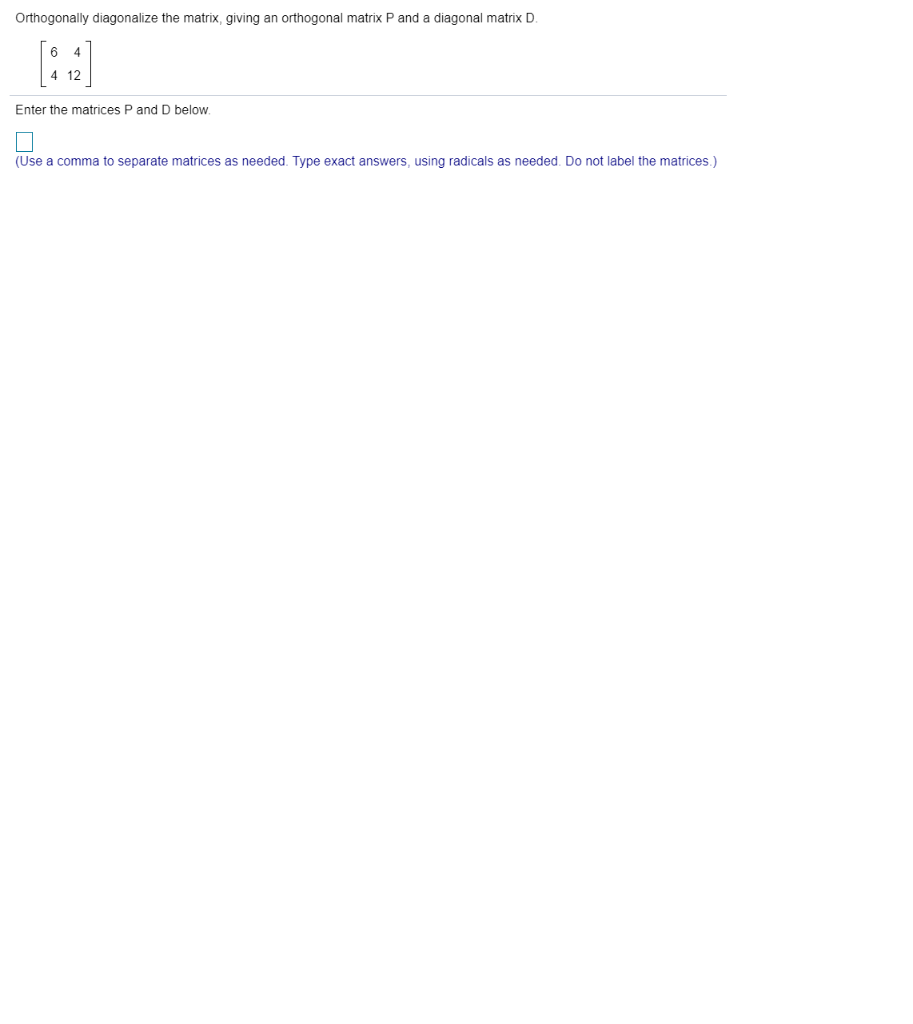Screenshot of a quiz question on orthogonal diagonalization. The task starts with the instruction, "Orthogonally diagonalize the matrix, giving an orthogonal matrix \( P \) and a diagonal matrix \( D \)." It is accompanied by a 2x2 matrix presented within brackets: [6, 4; 4, 12]. Students are instructed to enter the matrices \( P \) and \( D \) in a provided input field, which is currently empty. Below the input box, there is a blue note in parentheses stating, "Use a comma to separate matrices as needed. Type exact answers using radicals as needed. Do not label the matrices."